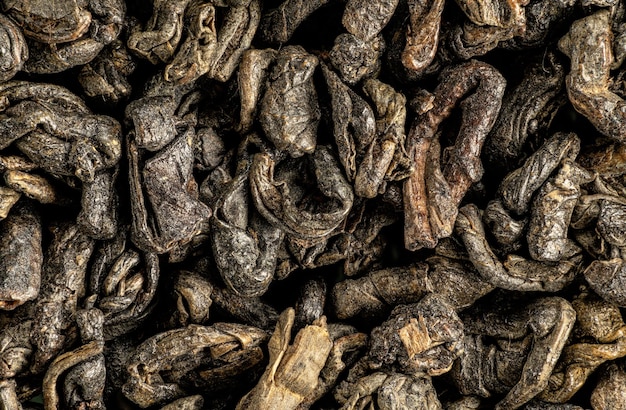The image portrays an abstract piece of artwork that can be interpreted as both a photograph and a painting, capturing textured, crumpled elements that evoke a sense of decaying organic matter. The canvas is dominated by varying shades of beige, brown, dark green, and black, creating a visually complex and somewhat unsettling array. These elements, resembling crumpled newspaper, woodchips, or even dried up cocoons, are intricately twisted and piled up, giving the appearance of either decaying leaves, old corn husks, or possibly even excrement. The textures are highly detailed, suggesting a 3D quality that might be more pronounced in person. The background remains faintly visible in black, adding depth and contrast. This dense assembly of rough, dirty-looking items spans the entire image, leaving the viewer uncertain whether it's a close-up of a larger mass or the complete pile itself. The artwork's ambiguity and rich textural complexity invite a multitude of interpretations, making it both intriguing and slightly disturbing.